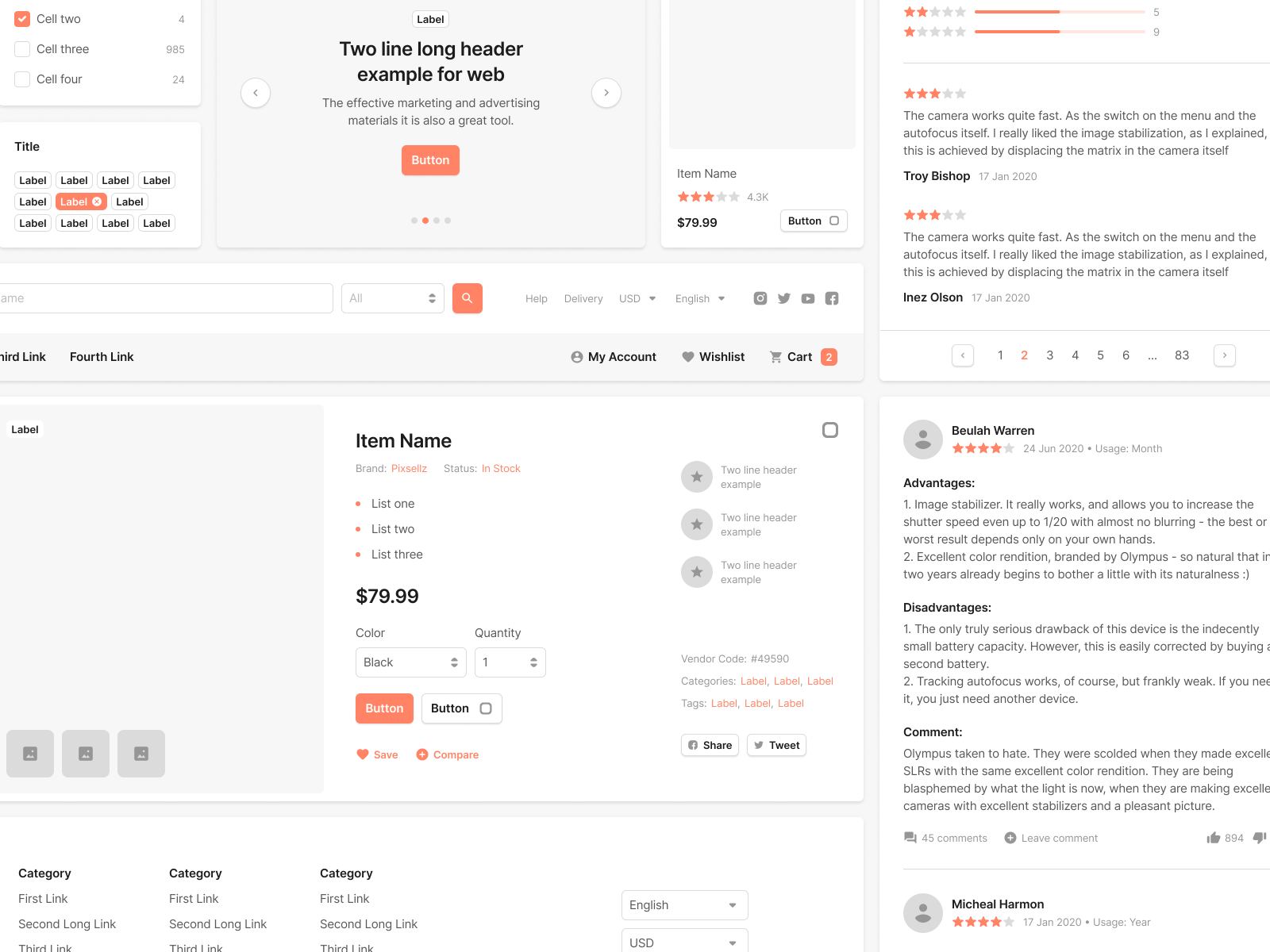This image depicts a product purchasing webpage with various interactive elements and detailed descriptions. 

In the top left corner, there is a selection box with multiple checkable options labeled as "Cell 2," "Cell 3," and "Cell 4," each accompanied by a white checkmark. Beneath this, there is a titling box, showcasing a highlighted label that also features a checkmark, indicating a selected option.

Towards the center, the header section spans two lines, featuring example text for web marketing and advertising materials. The header reads: "Effective marketing and advertising materials, it is also a great tool."

Below the header, an orange button stands out prominently. Adjacent to this button on the left side, there is a product description area, though it lacks an actual image. It lists an item name, accompanied by a 3-star rating, a price tag of $79.99, and a "hot button" for purchasing or further action.

On the far-right side, there is a section dedicated to menus or reviews, providing additional user insights or navigation options. 

Returning to the left side of the webpage, another product box is outlined. This box includes details such as an item name, a list of features (denoted as "List 1," "List 2," and "List 3"), the same price of $79.99, and fields to specify color and quantity.

Overall, the webpage design is organized and interactive, catering to a seamless product browsing and purchasing experience.